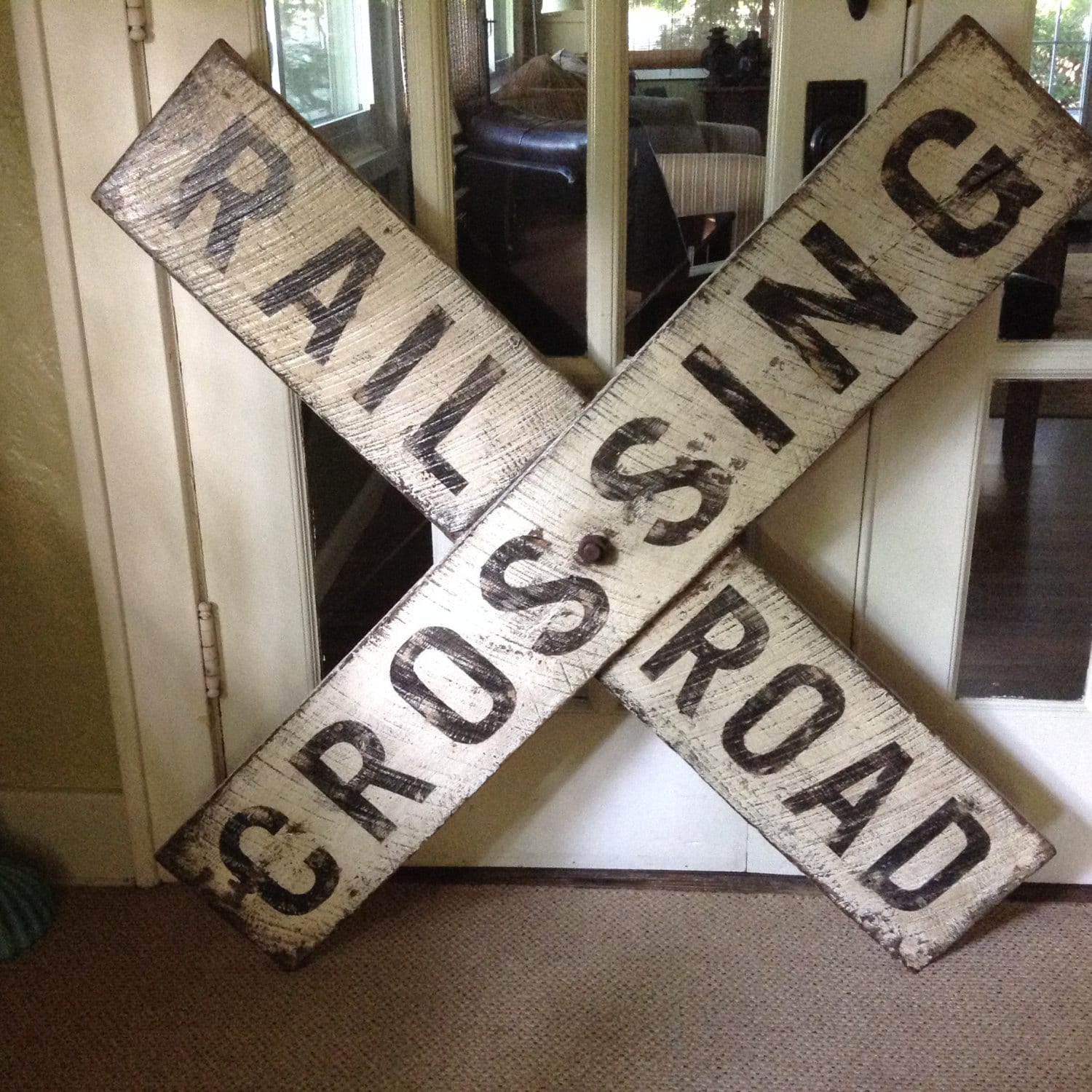In this image, a pair of white double doors form the focal point. These doors, adorned with glass windows offering a glimpse into another room containing chairs, a table, and outward-facing windows showcasing trees, are set against a light green or yellow wall on the left. Below the doors lies a light to greyish-brown carpet. Leaning against these double doors is an old, weathered railroad crossing sign, consisting of two white wooden planks forming an X shape. The plank angled from the bottom left to top right reads “Crossing” in black, faded text, while the one crossing it from the bottom right to top left displays the word “Railroad.” The sign, appearing aged and likely repurposed from an actual railway crossing, adds a nostalgic touch to the setting.